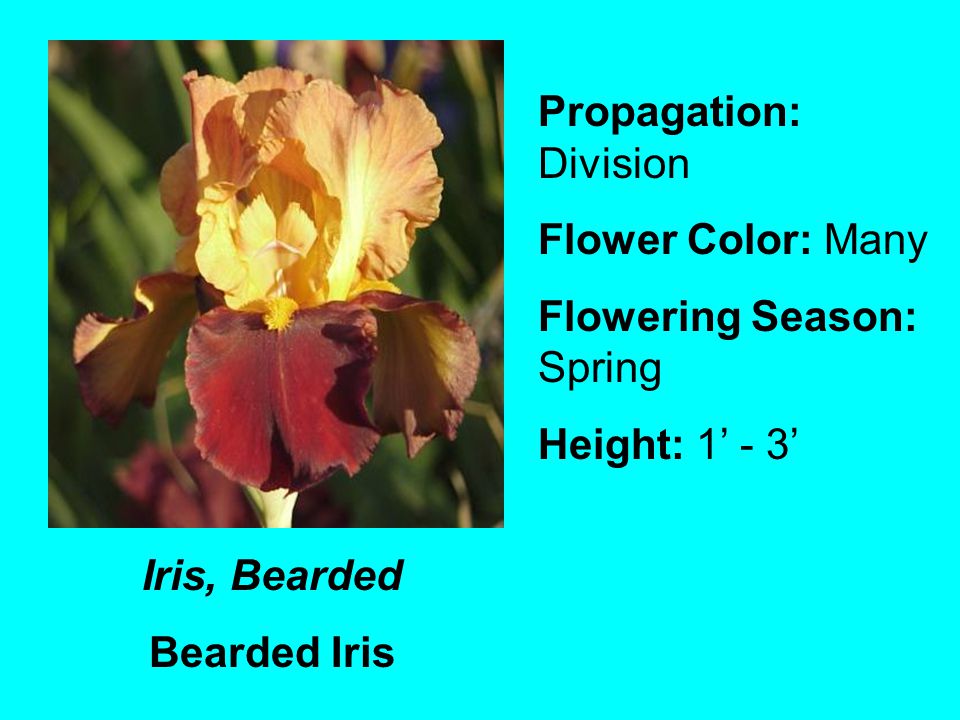The image has a bright light blue background and appears to be a slide from an educational presentation, possibly about botany. In the top-left corner, there's a detailed photograph of a bearded iris flower, with the label "iris, bearded" in italics below it, followed by "bearded iris" in black text. The flower displays multiple colors, including yellow petals predominantly pointing upwards and reddish petals hanging down. Surrounding the flower is a backdrop of green leaves or grassy area. To the right of the photograph, there is a list of text with bolded headers providing information about the plant: "Propagation: Division, Flower color: Many, Flowering season: Spring, Height: One foot to three feet." The text serves as an educational tool, potentially aimed at teaching about plant propagation and characteristics in a classroom setting.